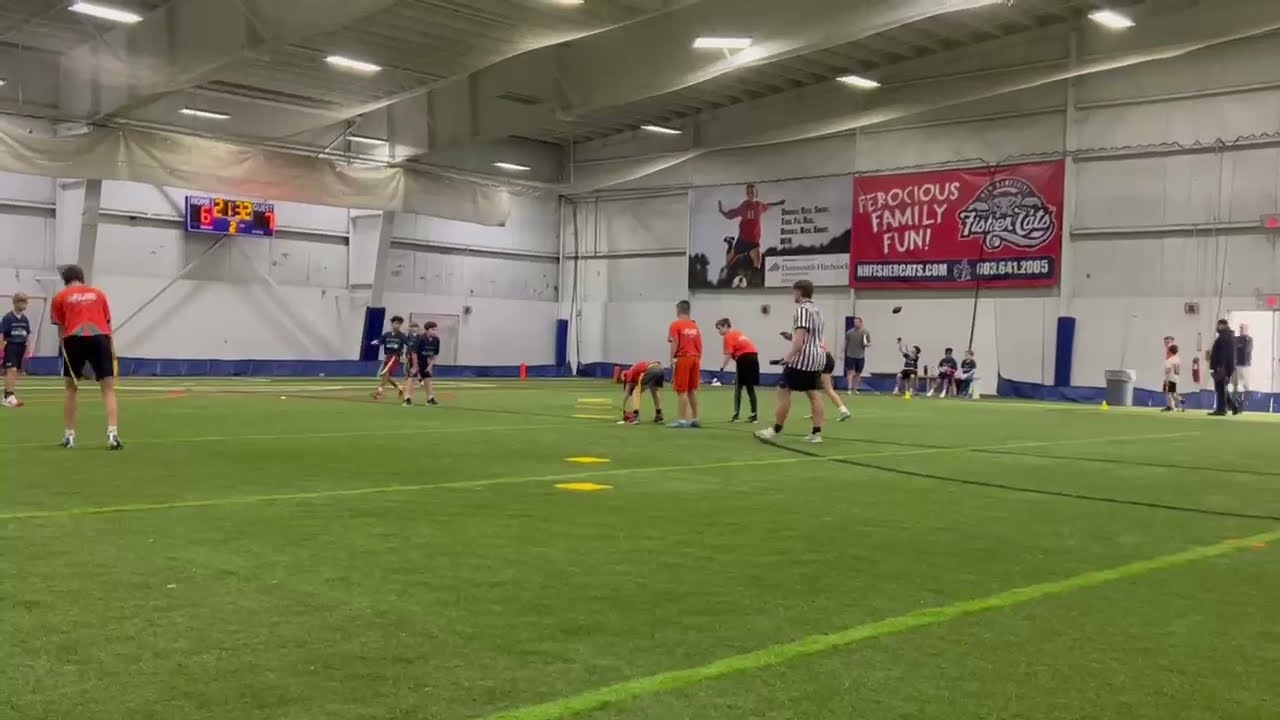The image captures a lively indoor soccer facility with a green artificial grass pitch. The setting is inside a large white metal building featuring an industrial-type ceiling with several lights. On the left side of the image, a team in blue uniforms can be seen, while a team wearing a mix of orange and black outfits occupies the foreground. Several young players, estimated to be between 10 and 15 years old, are in action on the field, with adults including a referee in black and white stripes and some coaches and parents in the background. 

The walls are adorned with various posters and signs. Notably, there's a large, vibrant sign with a red background and white text that reads "Ferocious Family Fun," accompanied by a logo resembling the Thundercats. Another sign on the left corner of the image displays a scoreboard with "Home 6," "21-52," and "Guest 7" in red. Additionally, a poster of a boy in a red shirt jumping is visible on the wall. Various equipment like cones and garbage cans are scattered around, and adults can be seen standing by, either watching the game or positioned at the entrance to the field. The uniformity of details, including colors and objects, creates a dynamic scene indicative of an engaging and well-organized sports event.